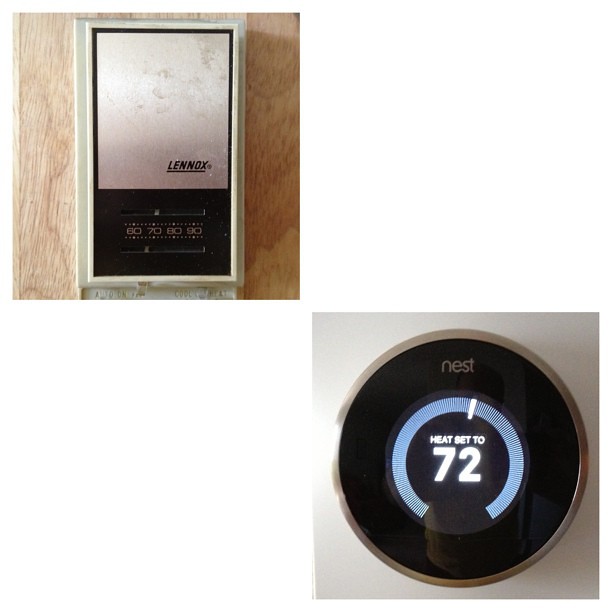In the image, the top left corner features a classic Lennox thermometer, devoid of any digital interface or touchscreen capabilities. This traditional device, likely many years old, has a simple design with two physical dials for regulating the temperature. In stark contrast, the bottom right corner showcases a modern Nest thermostat. This sleek, black, circular device boasts a touchscreen interface. It prominently displays "Heat Set to 72°F" in white text against a blue background. The highly reflective surface of the Nest thermostat captures the image of the person taking the photograph. The juxtaposition of the antiquated Lennox thermostat with the cutting-edge Nest device underscores the dramatic evolution of home climate control technology.